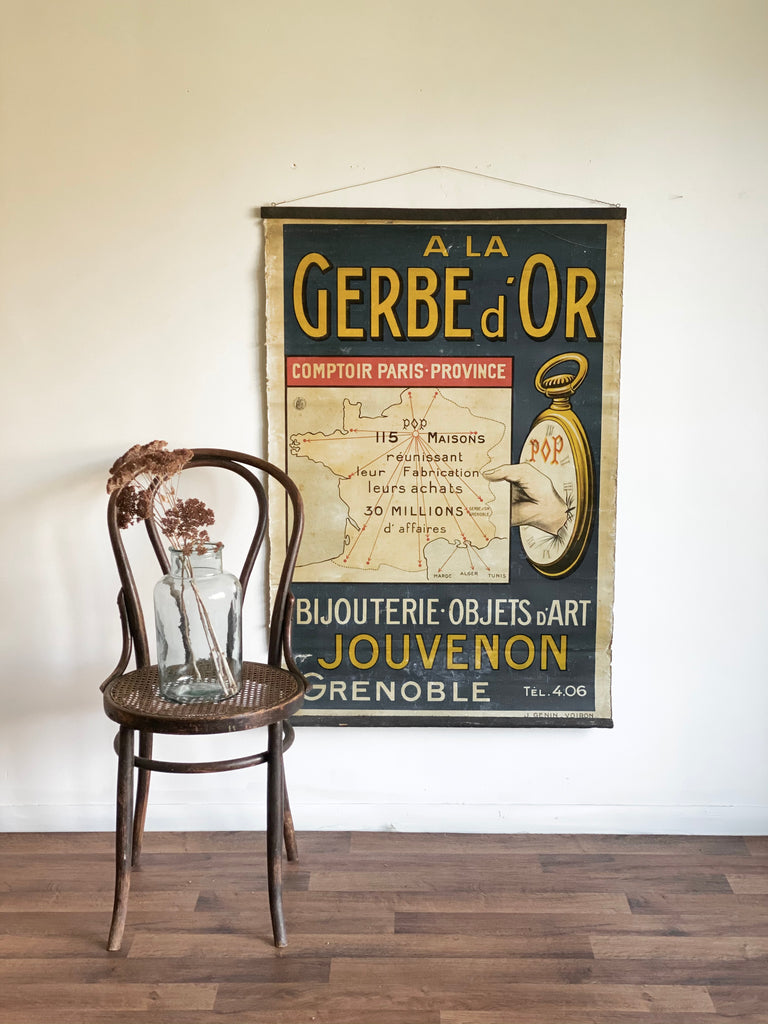In this image, a rustic wooden chair with thin legs and a rounded back sits on a floor that features a mix of dark and light brown hues. On the chair rests a clear mason jar vase filled with dried floral sticks, characterized by their brown stems and tops. The background wall is white, and a vintage French banner hangs from it, suspended by a thin black string, possibly attached to a nail. The banner's design includes black borders along its edges, with an off-white interior and a green backdrop. The banner is inscribed in French with various texts in yellow and white lettering, such as "A. La Guerbe d'Or," "Comptoir Paris Province," "Beaujolais Objects d'Art Jovenin Grenoble," and "Competitor Paris Province," among other phrases. A unique illustration features a hand emerging from a gold stopwatch with a white face, holding a piece of paper. The banner also includes a map of France, adorned with population information in black text.